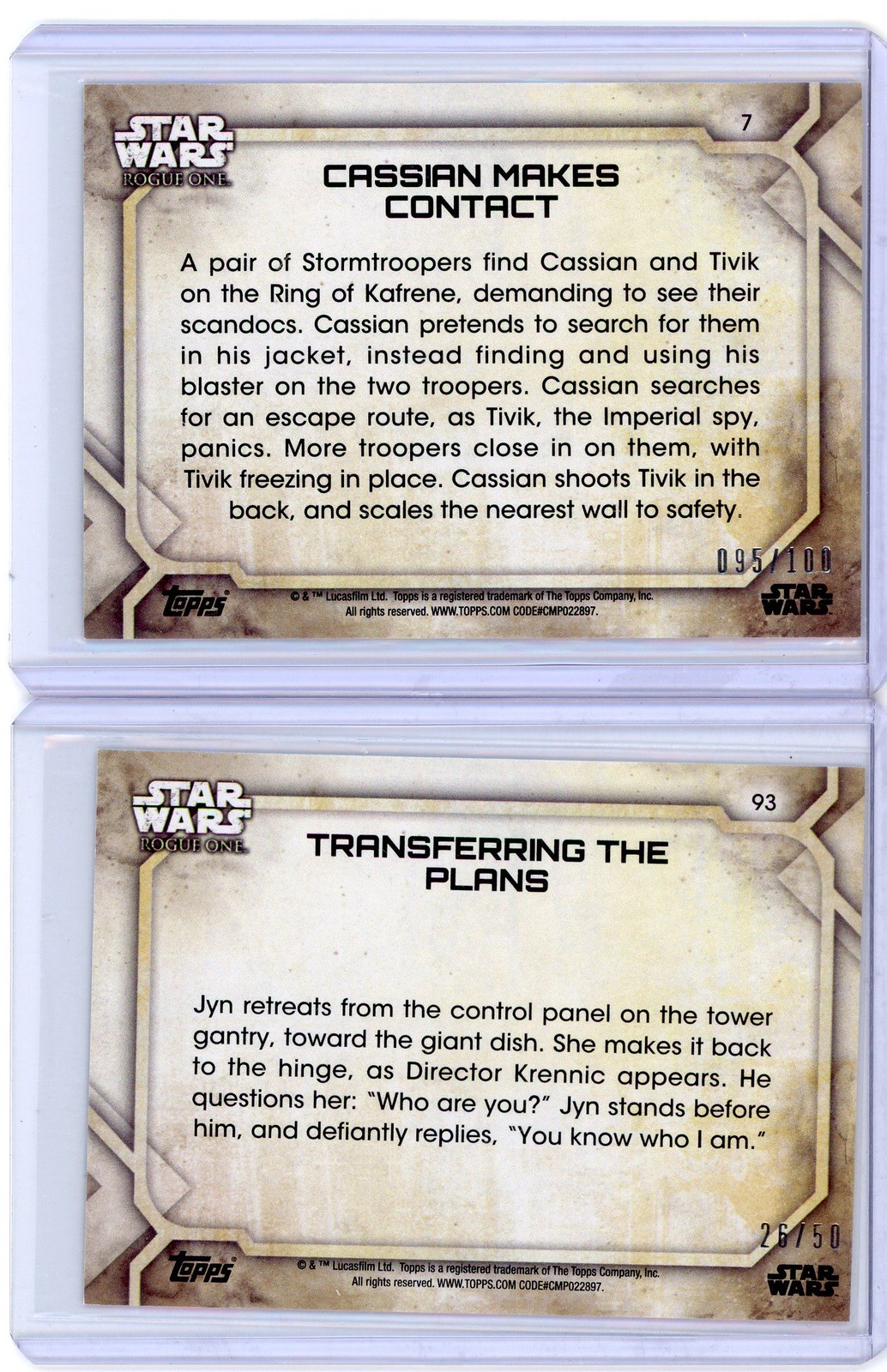This image depicts two Star Wars-themed playing cards in a white plastic laminated casing. Each card has an off-white, slightly dirty background that resembles a metal contraption. In the top left corner of both cards, it reads "Star Wars Rogue One" in white letters. The top card is titled "Cassian Makes Contact" in black letters and features a detailed narrative about a pair of stormtroopers finding Cassian and Tivek on the ring of Kafrene. They demand to see their set scan docs, but Cassian uses his blaster on the troopers and searches for an escape route while Tivek panics. More troops close in on them, and Cassian ultimately shoots Tivek in the back before scaling a wall to safety. The bottom card is titled "Transferring the Plans" in bold, all-capital black letters. It narrates Jyn's retreat from the control panel on the tower gantry toward a giant dish, her confrontation with Director Krennic, and her defiant reply, "You know who I am." In the bottom right corner of each card, "Star Wars" is printed in black letters, providing additional branding. The cards are possibly being preserved in a collection, stored in this protective casing, potentially due to their worth or value.